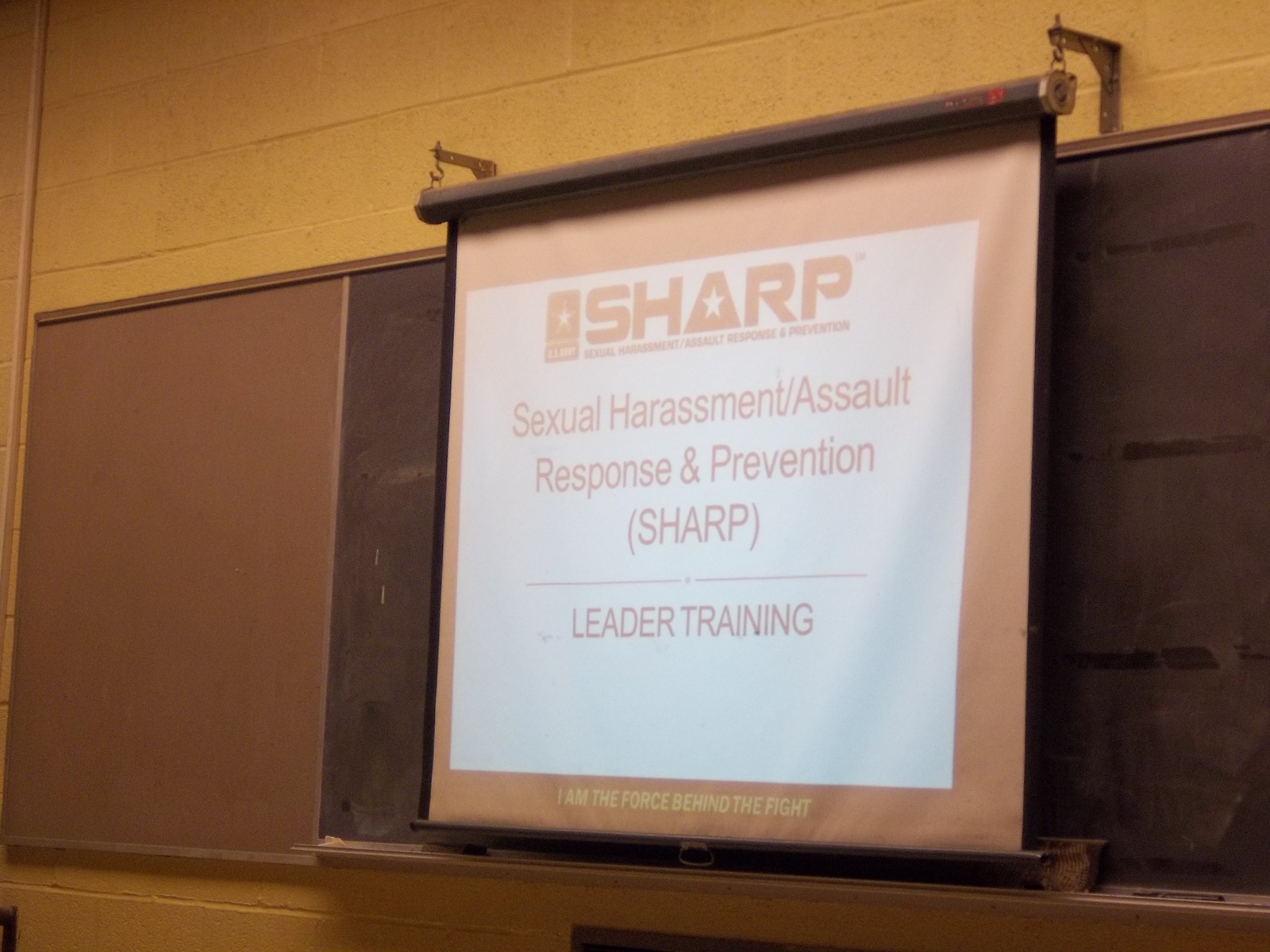In the image, there is a photograph of a somewhat dimly lit and old classroom. A projector screen is prominently displayed, pulled down in front of a well-worn black chalkboard that has some marks and dirt on it. The screen is mounted to a white painted brick wall, and the brackets securing it are visibly screwed into the wall. The screen itself displays a PowerPoint slide with a white background and a peach-colored border.

At the top of the slide, there is a logo accompanied by the text "SHARP," which stands for "Sexual Harassment/Assault Response and Prevention." Directly below that, in parentheses, it reiterates "SHARP." Beneath this, a dividing line separates the main title from the subheading, "Leader Training." At the bottom of the slide, within the peach border, it reads, "I am the force behind the fight." To the left of the image, there is a section of brown slate, similar in texture to the chalkboard but distinct in color.